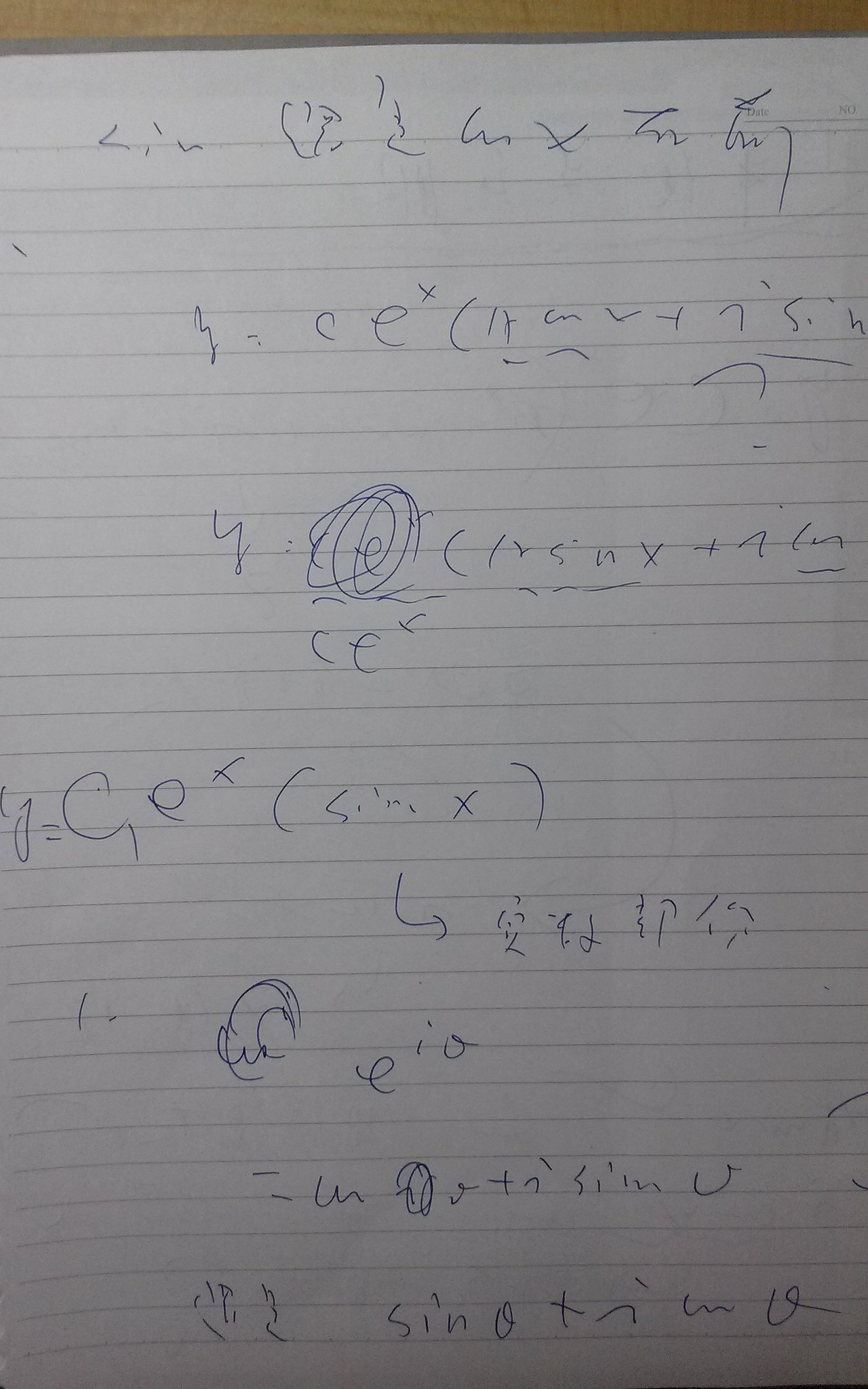The image displays a piece of white lined paper filled with hastily scribbled mathematics equations, characterized by extremely illegible handwriting. The majority of the content is difficult to decipher, with some elements resembling random symbols. At the top-middle of the page, part of an equation is obscured by a large spiral scribble, making it impossible to read what's underneath. Visible fragments nearby include the partial words or letters "F-E-R" and "C-E," with the latter crossed out and rewritten.

On the top row, the notation "L-I-N" is followed by several unidentifiable symbols and the letter "X." The second row also contains a mix of unreadable symbols and the expression "E^X" followed by parentheses enveloping additional symbols, culminating in "SIN" at the row's end. Below this, the equation continues with a "Y" and the previously mentioned crossed-out symbols, trailed by more parentheses enclosing "S-N-X-T-A-L-N."

Further down, the paper shows "Y equals G-E-X," encapsulated in parentheses, followed by "SIN-X." An arrow descends from this equation, pointing to even more illegible symbols, which increasingly clutter the space towards the bottom of the page. Despite the chaotic scribbles, recognizable fragments like "SIN," "T," and "N" sporadically appear among the indecipherable content.